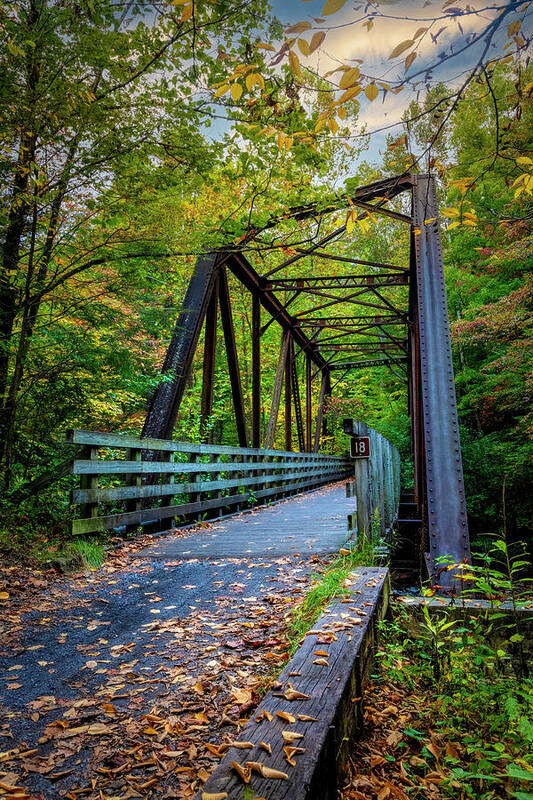The image captures a picturesque footbridge located in a wooded forest area during early fall. The wooden bridge, designed for pedestrians, features a metal grid tower structure with vertical beams that rise roughly 15-20 feet, interconnected with zigzagging metal bars across the top, allowing an unobstructed view of the sky and surrounding trees. On either side of the bridge are wooden railings, and prominently displayed on the right-hand railing is a distinctive sign - a brown square bordered with yellow and marked with the number 18 in red.

The scene is richly imbued with autumnal hues: the pathway leading to the bridge is blanketed with a mosaic of leaves in shades of brown, yellow, orange, and hints of green. Trees flanking the bridge exhibit a similar gradient of fall colors, under a blue sky with scattered clouds. This tall, lengthy bridge elegantly traverses the forest floor, encapsulating the serene and vibrant essence of the fall season.